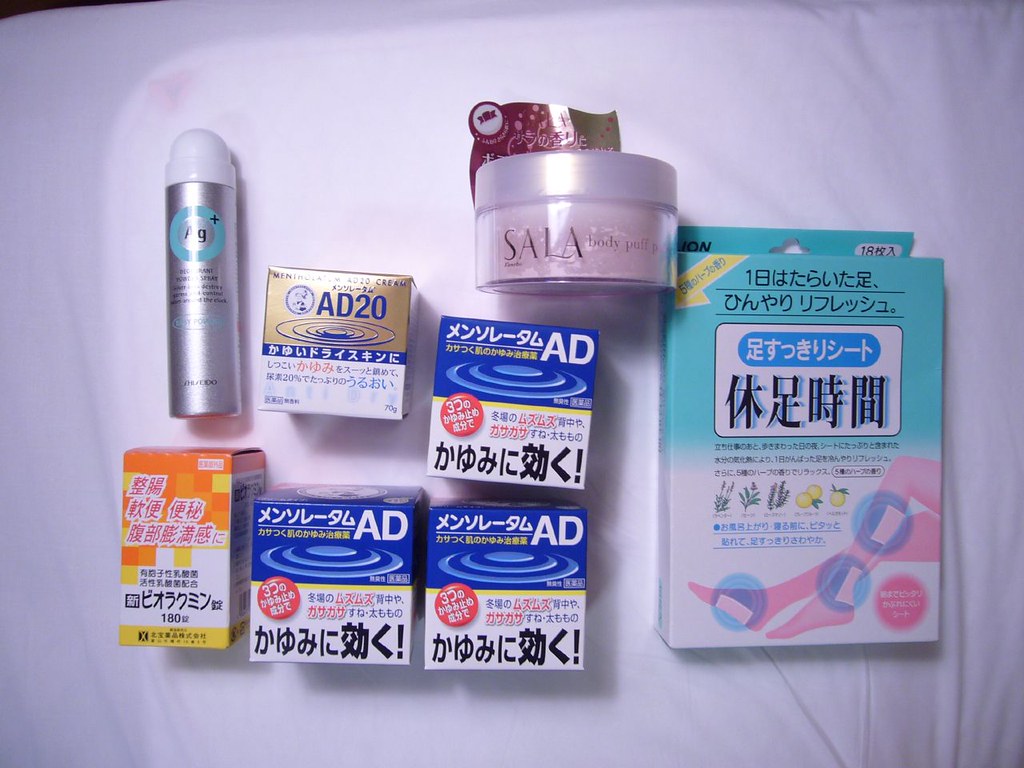This image, captured from a bird's-eye view, showcases an assortment of nine distinct boxed products arranged neatly on a white tablecloth. All the packages feature text in an Asian language, likely Japanese. 

Among the items, three are identical blue and white boxes labeled "AD." They form an 'L' shape with two horizontally aligned and one positioned vertically above them. Each of these boxes has a blue upper half and a white lower half.

Adjacent to these is another box-shaped item with a gold upper section and a white lower section. Nearby, you can also see a vertically oriented rectangular box, featuring an orange top half and a white bottom half, breaking the color pattern seen in the "AD" boxes.

Above this orange and white rectangular box is a cylindrical product, possibly a deodorant, with a silver body, black text, and some blue accents. Positioned more towards the right side of the image and above one of the blue and white "AD" boxes, there’s a pink and silver item labeled as a "solid body puff."

To the far right of the arrangement stands a larger product, characterized by light blue, blue, and white packaging. This box is unique in design, displaying an image of two legs with blue cooling pads.

All these varied items, still sealed in their respective boxes, are meticulously placed on a table covered with a pristine white cloth.